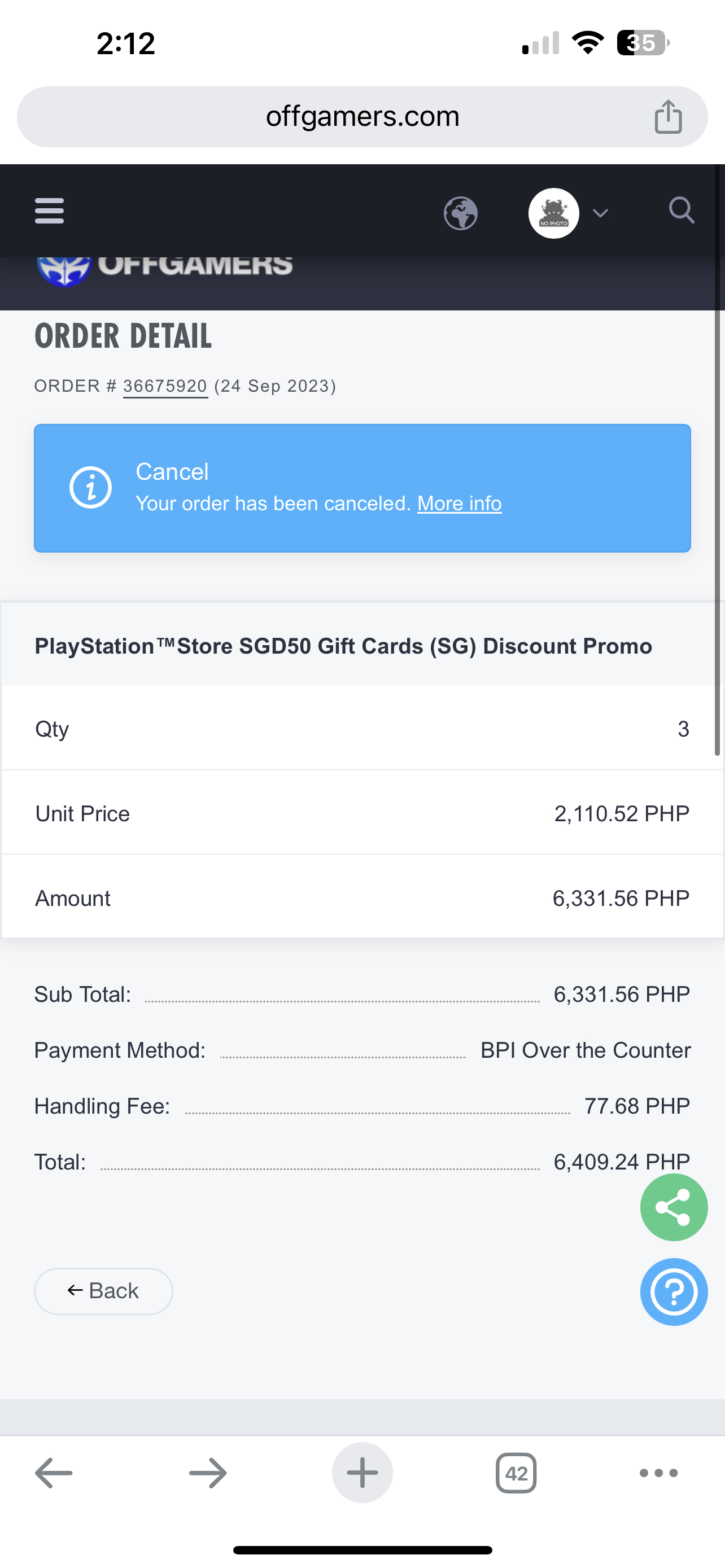The screenshot depicts a transaction summary from the website 'OffGamers'. At the top, the browser window displays "Off Gamers", with a right-side icon showing a square with an upward-pointing arrow. In the top left corner, there is the number '212' and the battery level is at 35%. The Wi-Fi signal is full, but the cellular signal shows only one out of four bars.

Below the browser bar, there's a black bar featuring a hamburger menu icon (three horizontal lines) and a globe icon. Underneath, "OffGamers" appears again along with the heading "Order Detail" and an order number, which appears partially readable as '3...4'. The date is marked as 24th September 2023.

A blue rectangle contains an eye icon and the word 'Cancel', indicating the order's cancellation status, accompanied by the text "Your order has been cancelled" and an underlined "More info".

Further down, the order details list a "PlayStation Store SGD50 gift card" (SGD Discount Promo), with a quantity of three. The unit price is 2,110.52 PHP, summing to an amount of 6,331.56 PHP. The subtotal is also 6,331.56 PHP. The payment method indicated is "BPI Over-the-Counter", with a handling fee of 77.68 PHP, making the total 6,409.24 PHP.

At the bottom of the screen, there is a green circle with a share button, a blue circle with a question mark inside, and a back button. There are also navigation arrows (left and right), a plus sign, a square icon, and a number '42' centered. The bottom of the image shows a black bar.